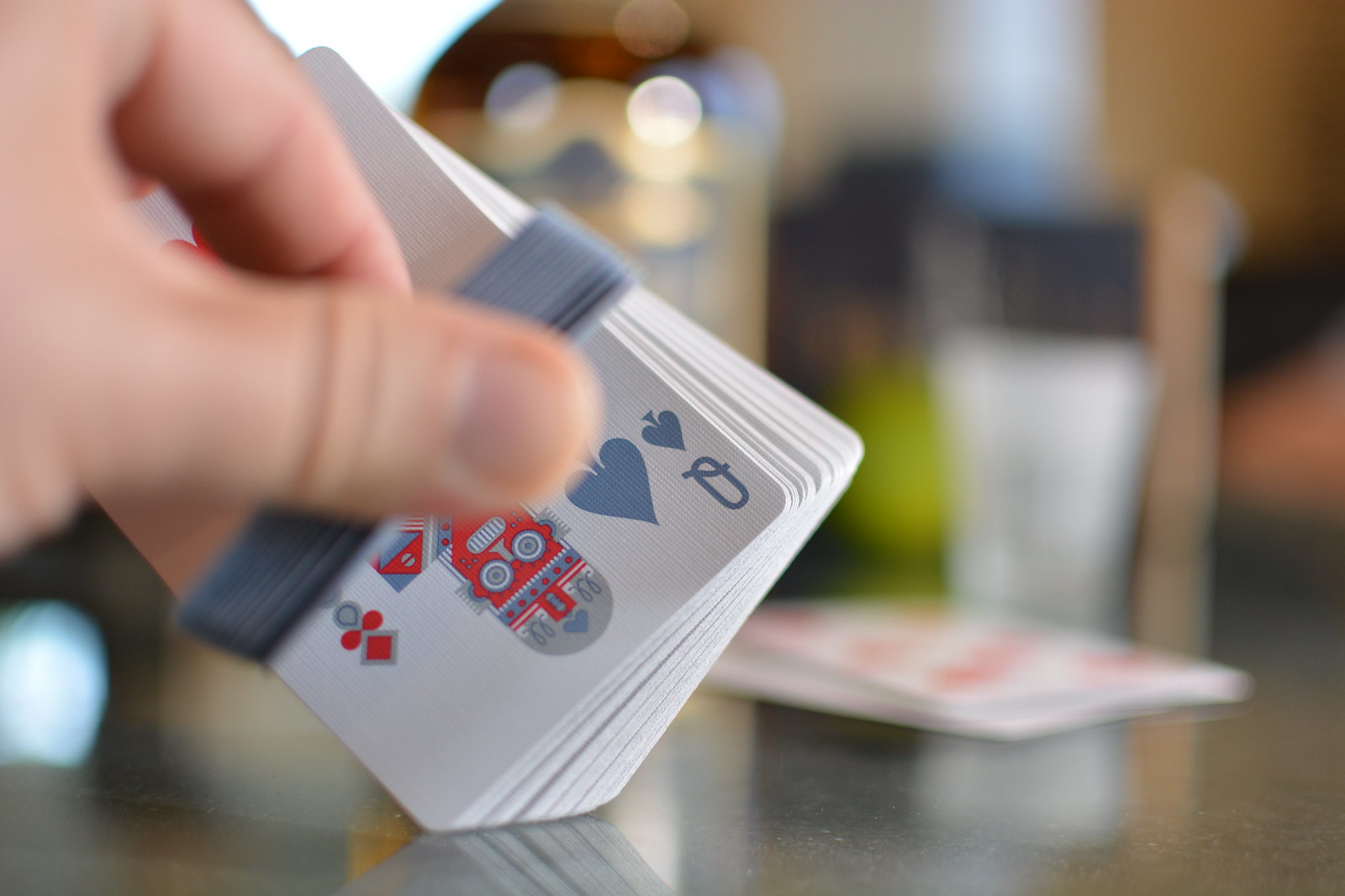The image captures a focused view of a deck of cards in the foreground set within an indoor room. The background is artistically blurred, creating an impressionistic scene that includes a cylindrical object adorned in yellow and blue hues to the left, while to its right appears a white cup-like item. Spread out on the grayish, almost stone-like tabletop are additional playing cards lying face up. Emerging from the left side of the frame is a white hand, thumb and index finger discernible, grasping the deck of cards secured by a gray band. The deck's visible bottom card is a unique Queen of Spades, depicted in a striking silver color. This Queen diverges from traditional imagery, resembling a robot with a semicircular gray head adorned with vibrant shapes and colors. Her red robotic face features circular eyes, topped with a blue band decorated with small red circles, adding a futuristic flair to this classic card game.